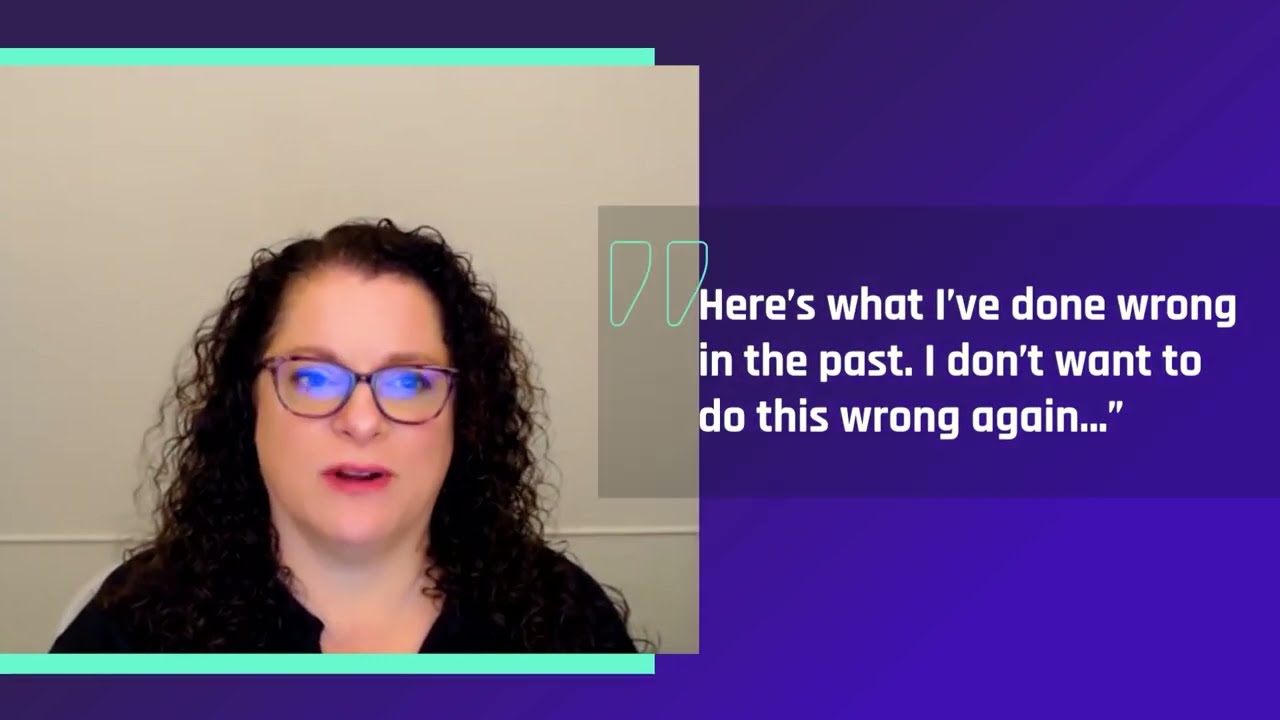The image features a woman with pale skin, long curly dark hair cascading past her shoulders, and brown-framed glasses, who appears to be wearing a black shirt and pink lipstick. She looks directly at the viewer with her mouth slightly open, as if speaking. She is placed within a picture frame with a light turquoise border at the top and bottom. The background of the image is predominantly purple with a blue outline. To the right of the woman, against the purple background, there is a prominently displayed quote in white font: "Here's what I've done wrong in the past. I don't want to do this wrong again..." The quote is lightly adorned with painted or cartoon-like quotation marks in blue, adding a stylistic touch. The image is solely focused on the woman and the quote, with no other individuals or additional text present.